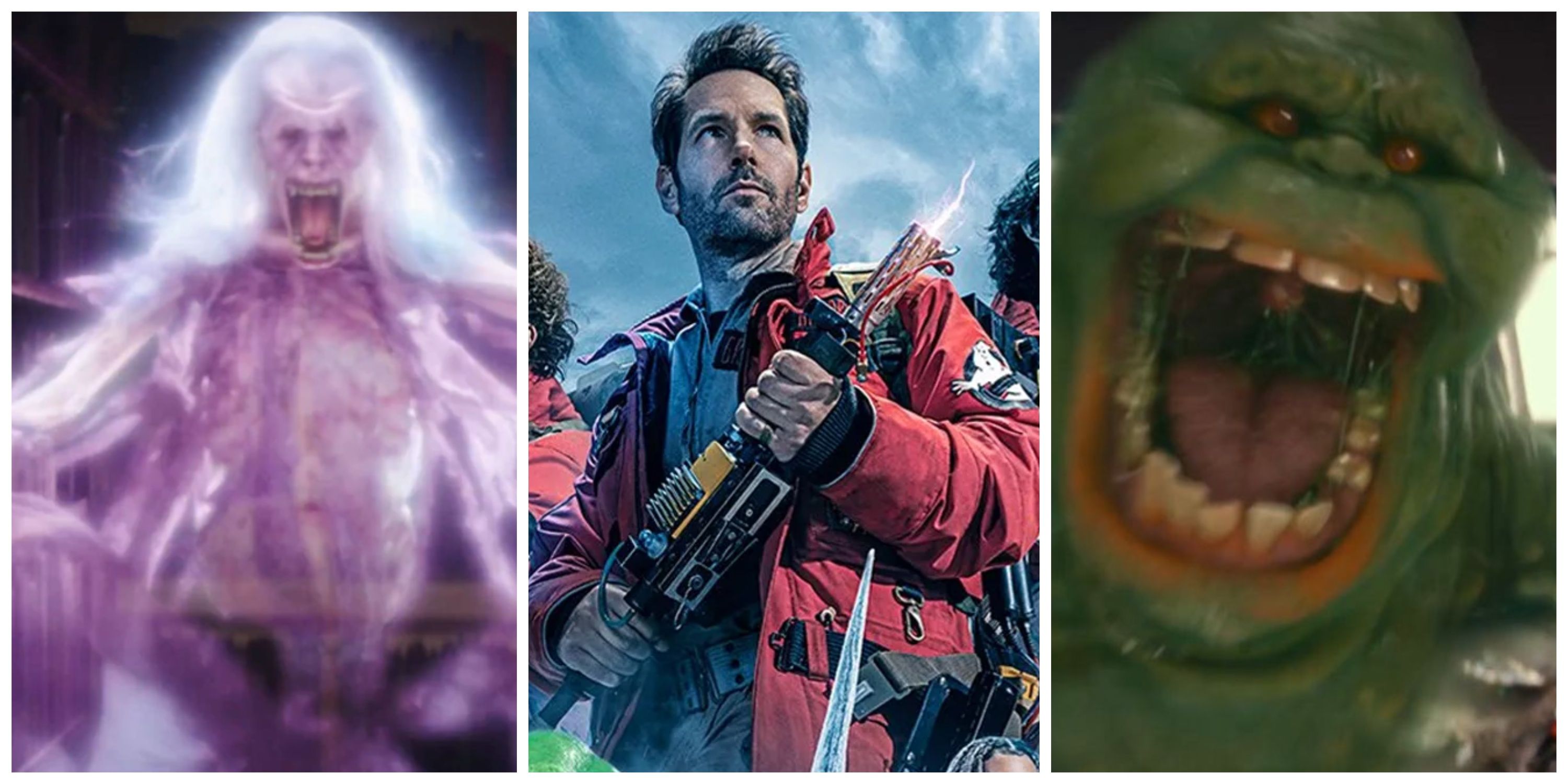The image is a horizontally rectangular composition made up of three equal-sized, full-color photographs from the movie "Ghostbusters," each separated by thin vertical white lines. On the left, there is a screen grab of a semi-transparent, 3D generated ghost with a humanoid appearance. This ghost has a skeleton-like face, a wide-open mouth showcasing large yellow fangs and a large pink tongue, and long white hair. The central photograph features a man, presumed to be Ryan Reynolds, gazing up to the top right. He is dressed in a red overcoat and a tan jumpsuit, and he is holding a futuristic sci-fi gun emitting a white bolt of lightning. The image on the far right is another 3D generated ghost, a greenish creature resembling a fat slug without legs, characterized by its large mouth filled with human-like teeth. The overall effect is a vivid, detailed triptych capturing dramatic moments from the film.